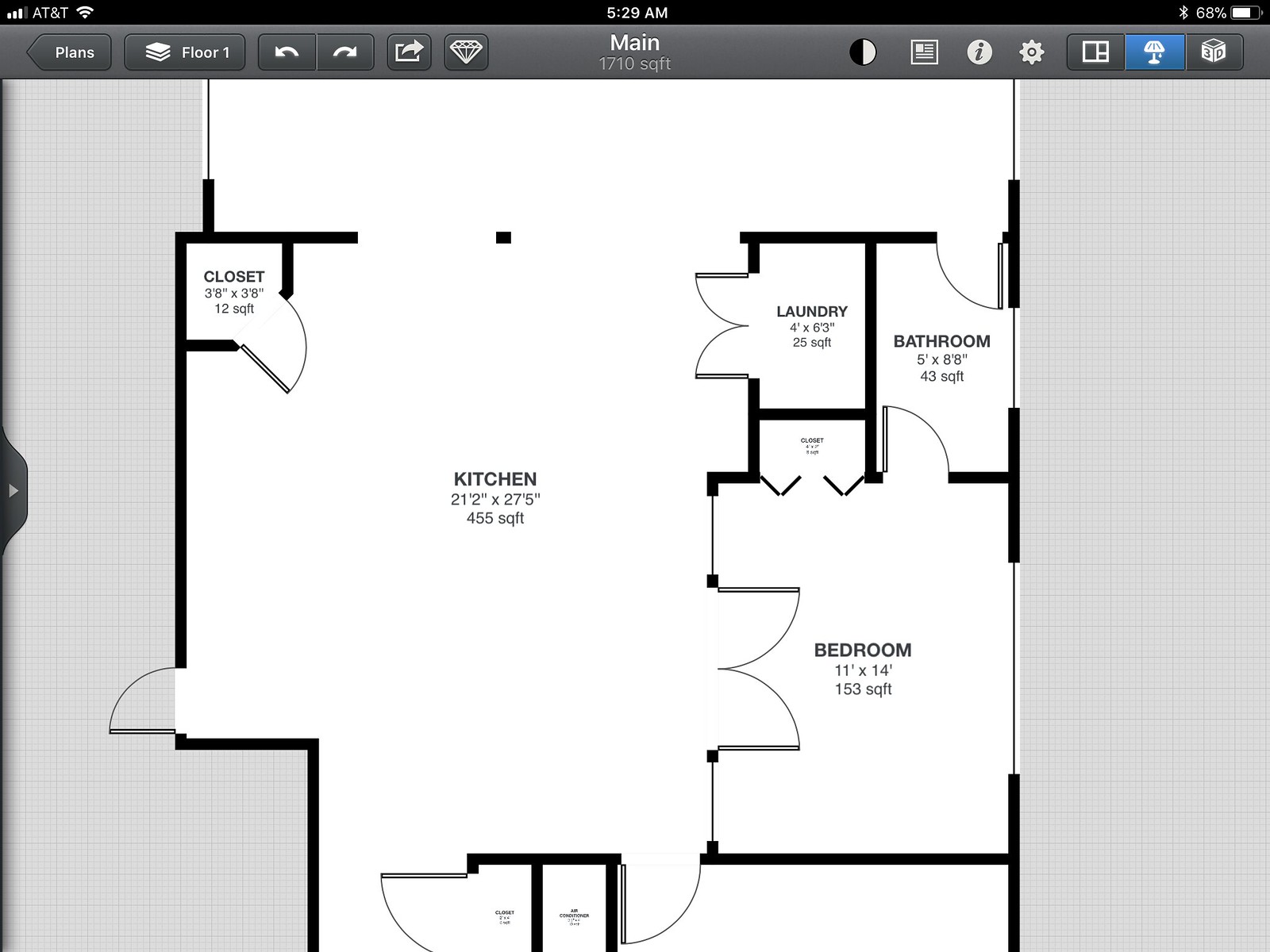The image appears to be a screenshot of a digital floor plan displayed on a device, likely a smartphone or tablet, as indicated by the AT&T label at the top. The time shown is 5:29 AM. The floor plan covers a segment of a house totaling 710 square feet, showcasing specific rooms and key features.

At the bottom right of the image, an exterior door leads directly into a spacious kitchen that measures 21 by 27 feet. Within the kitchen, there is a designated closet area. Adjacent to the kitchen, a laundry room is positioned, providing a functional space for household chores. Additionally, a bedroom is accessible from the kitchen, and this bedroom features an attached bathroom. The bathroom is equipped with two entry points: one from the bedroom and another leading to an unspecified room at the top of the floor plan.

The top portion of the floor plan, while not fully detailed, contains areas yet to be labeled or identified. Small closets can be seen towards the bottom of the image. The image seems to capture only a middle section of the entire floor, excluding the front door and other potential bedrooms or spaces that may exist elsewhere in the design.

The top of the image includes a navigational bar with the label "Plans Floor 1," suggesting this is the first level of a multi-story home. Overall, the floor plan offers a glimpse into the layout and design of a portion of the house, hinting at further details available on the complete digital display.